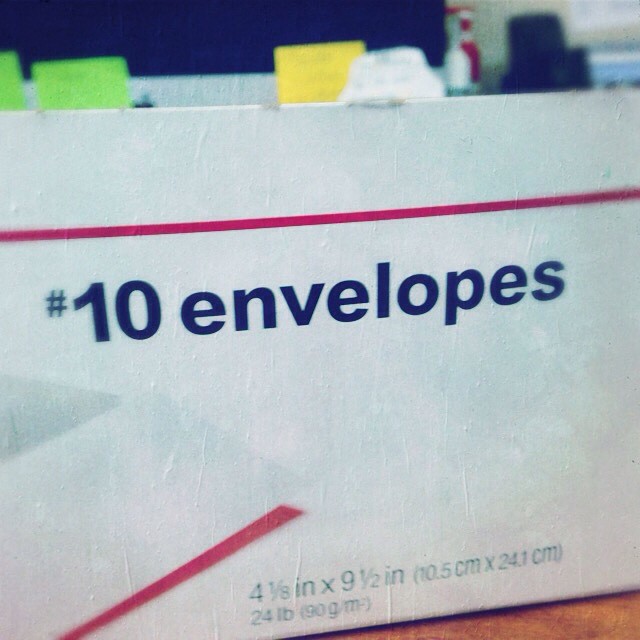This detailed close-up photo focuses on a white box of Number 10 envelopes, prominently featuring a thin pinkish-red stripe near the top. Bold, blue text across the front reads "#10 Envelopes." Lower on the box, dimensions are stated: "4 1/8 inch x 9 1/2 inch" followed by "10.5 cm x 24.1 cm" in brackets, alongside "24 LB (90 G/M2)." 

Part of an envelope is displayed on the front for reference. In the background, the image is out of focus but reveals hints of an office setting; yellow and green Post-it notes are visible, alongside what might be a desk and other office supplies. A small part of a brown table is also seen at the bottom right corner. The backdrop consists of a white wall with some indistinct blue elements and a metallic feature, likely contributing to the office ambiance.